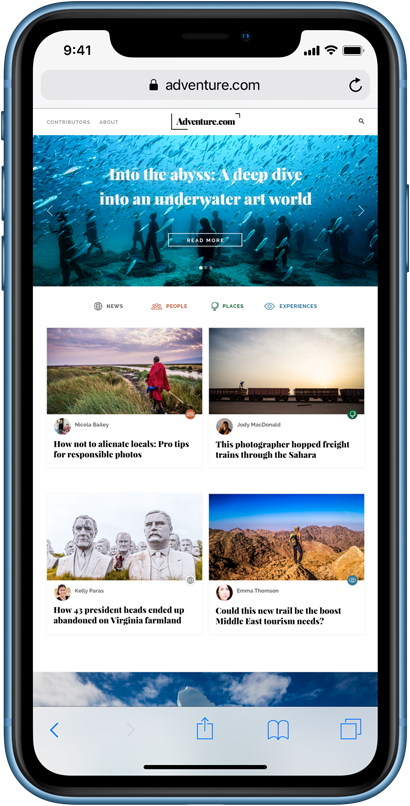This is an image of a smartphone's front display. The device shows a fully charged battery, full Wi-Fi signal, and strong cellular reception, with the time displayed as 9:41 AM in the top left corner. The screen is currently displaying a web page from adventure.com.

At the top of the webpage, the site's logo "adventure.com" is prominently displayed, flanked by navigation menu options on the left—such as "Contributors" and "About"—and a search icon on the right. Below this header, a striking cover photo spans the full width of the screen. The image features underwater statues surrounded by swimming fish, with an overlay of white text that reads, "Into the Abyss: A Deep Dive into an Underwater Art World." A "Read More" button is positioned below this heading.

Beneath the cover photo are four clickable categories in different colors: "News" (gray), "People" (orange), "Places" (green), and "Experiences" (blue). Following these categories, four article previews are displayed with respective images and titles:

1. "How Not to Alienate Locals: Pro Tips for Responsible Photos" accompanied by a picture of a person in a red coat walking through a grassy field.
2. "This Photographer Hopped Freight Trains Through the Sahara" paired with an image of a train traversing a desert, featuring someone standing atop one of the train cars.
3. "How 43 Presidents' Heads Ended Up Abandoned on Virginia Farmland," illustrated with a striking image of stone busts of Presidents Lincoln and FDR.
4. "Could This New Trail Be the Boost Middle East Tourism Needs?" alongside a photograph of a woman standing on a brown mountain, overlooking a vast terrain.